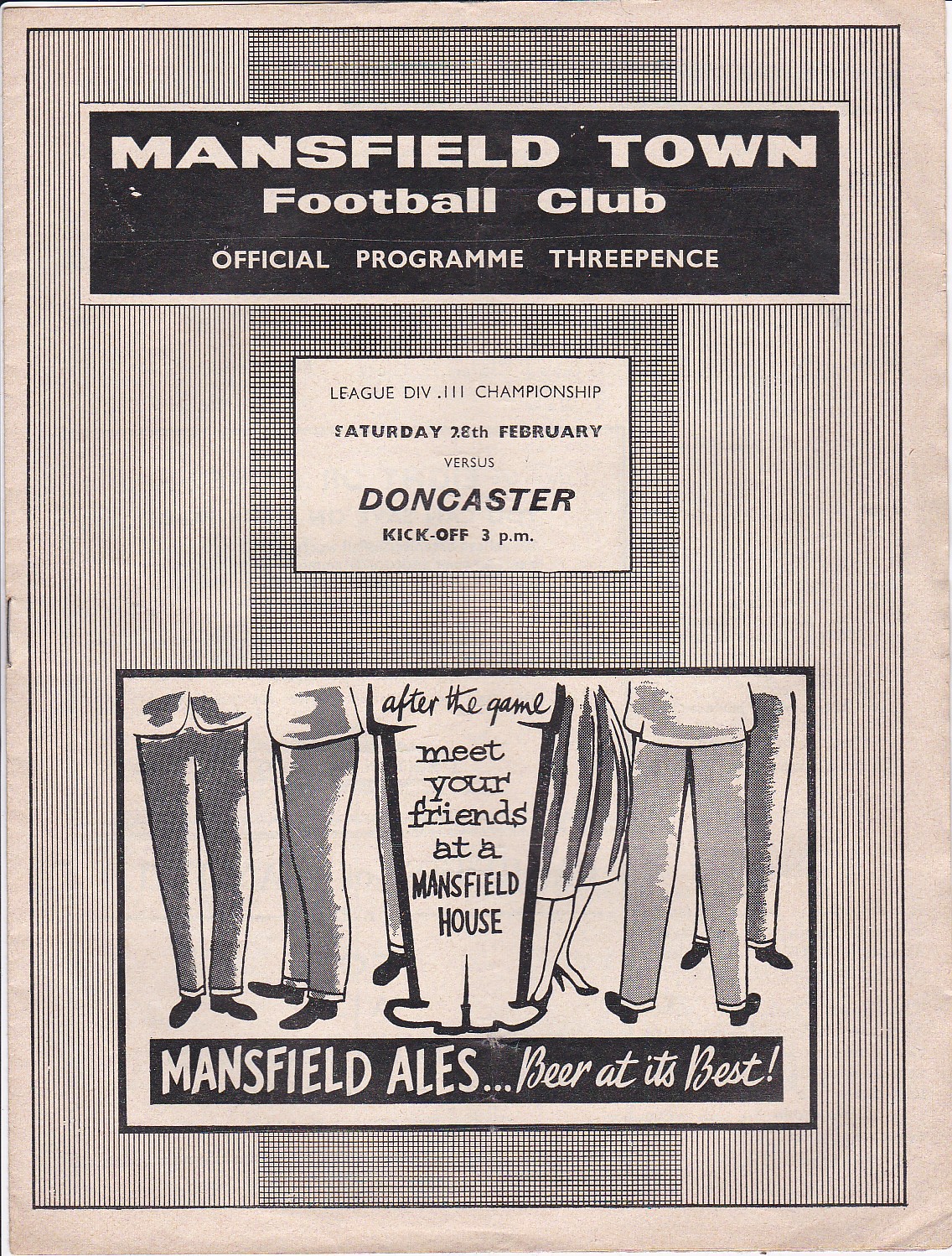This image depicts an old-school program for a British football game, emanating a vintage charm with its tan and beige paper, presented entirely in black and white. At the top of the image, a black banner with a white outline prominently displays "Mansfield Town Football Club, Official Program, Three Pence." Directly beneath this banner, a white box with a black outline details the game specifics: "League Division III Championship, Saturday, February 28th versus Doncaster, Kickoff, 3 p.m.," with the words "Doncaster" and "kickoff" highlighted in bold. The background of the image features a pattern of vertical lines, with the middle section characterized by a crosshatch design of intersecting horizontal and vertical lines. Towards the bottom, a black and white photograph captures the lower halves of several men and women, emphasizing their legs and feet. Amidst this image, a caption encased in a white outline reads, "After the game, meet your friends at Mansfield House." Below this, another black banner proudly states, "Mansfield Ales, beer at its best."